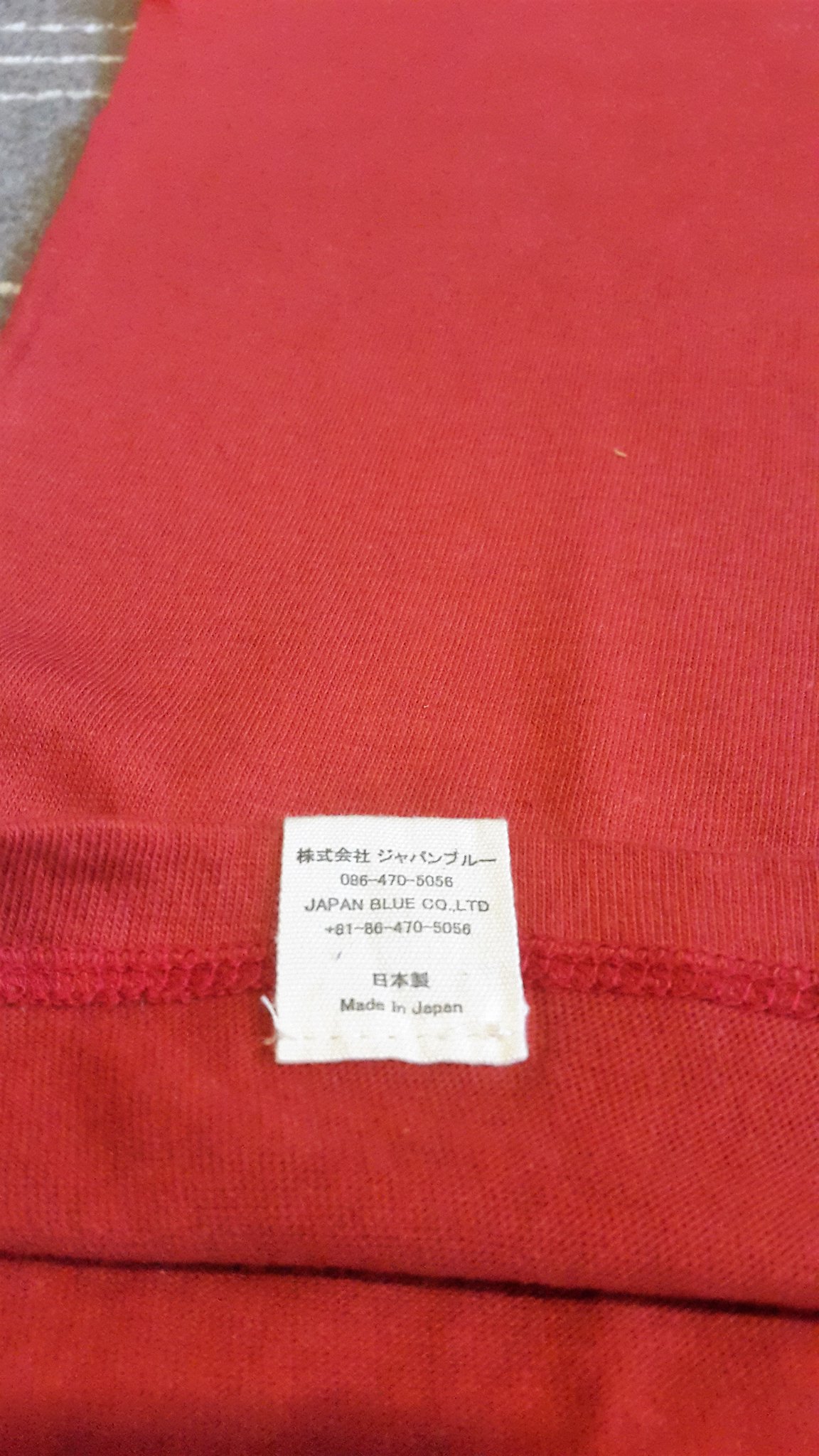This image features a neatly folded red shirt adorned with a small white tag. The tag displays black writing in multiple lines. The top line consists of text in an unfamiliar language. Beneath it, the second line includes the numerical sequence "086-470-5056". The third line reads "Japan Blue Company Limited," followed by "61-86-470-6056" on the fourth line. Several lines down, more characters in a different, unrecognized language appear. The final line of the tag states "Made in Japan." The shirt is set against a backdrop of gray fabric, which is detailed with white stitching in straight lines.